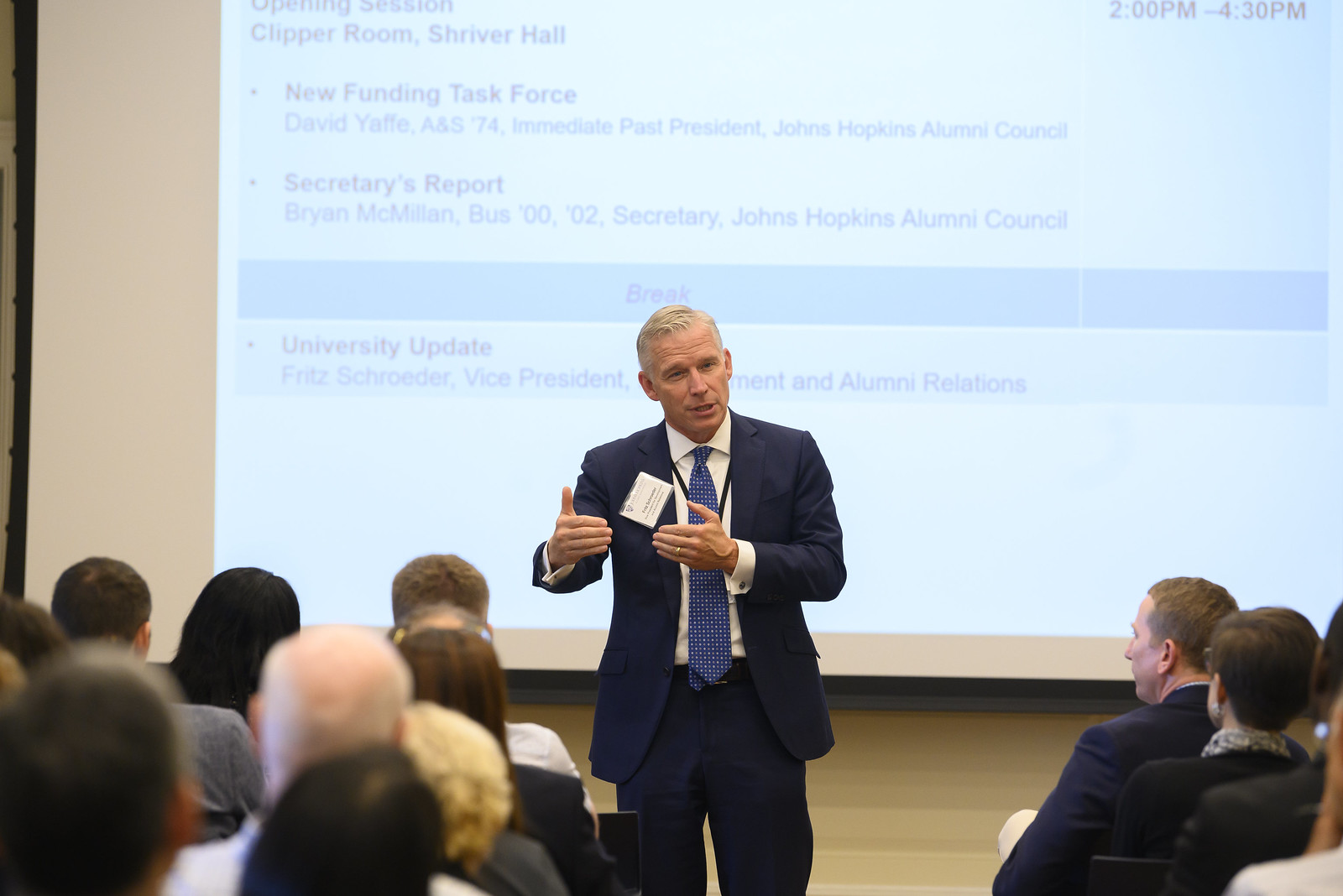This image captures a detailed scene of a lecture presentation. In a spacious room filled with attentive audience members, a distinguished man stands at the center, giving a compelling presentation. He is positioned towards the bottom-center of the image, dressed impeccably in a dark blue suit paired with a white button-up shirt and a blue tie adorned with tiny white polka dots. His gray hair is slicked back, and he has a name label attached to the right side of his jacket. He appears animated, gesturing with both hands raised, palms facing him, and wearing an expressive look.

Behind the speaker is a large white projection screen that dominates most of the wall, bordered in black. Projected onto this screen is a PowerPoint slide with a light gray background, displaying various text details. At the top left, the slide reads: "Opening Session, Clipper Room, Shriver Hall." Following this title, several bullet points list session details: "New Fundings Task Force, David Yaffe, ANS, '74, Immediate Past President, John Hopkins, Alumnae Castle," and "Securities Report, Brian McMillan, BUS, '0002, Secretary, John Hopkins, Alumnae Castle."

Rows of attendees can be seen seated, captured from an audience member's perspective, with the backs of their heads visible in the foreground, all focused intently on the speaker's lecture. The immersive setup and detailed visual elements convey a lively and engaging presentation atmosphere.